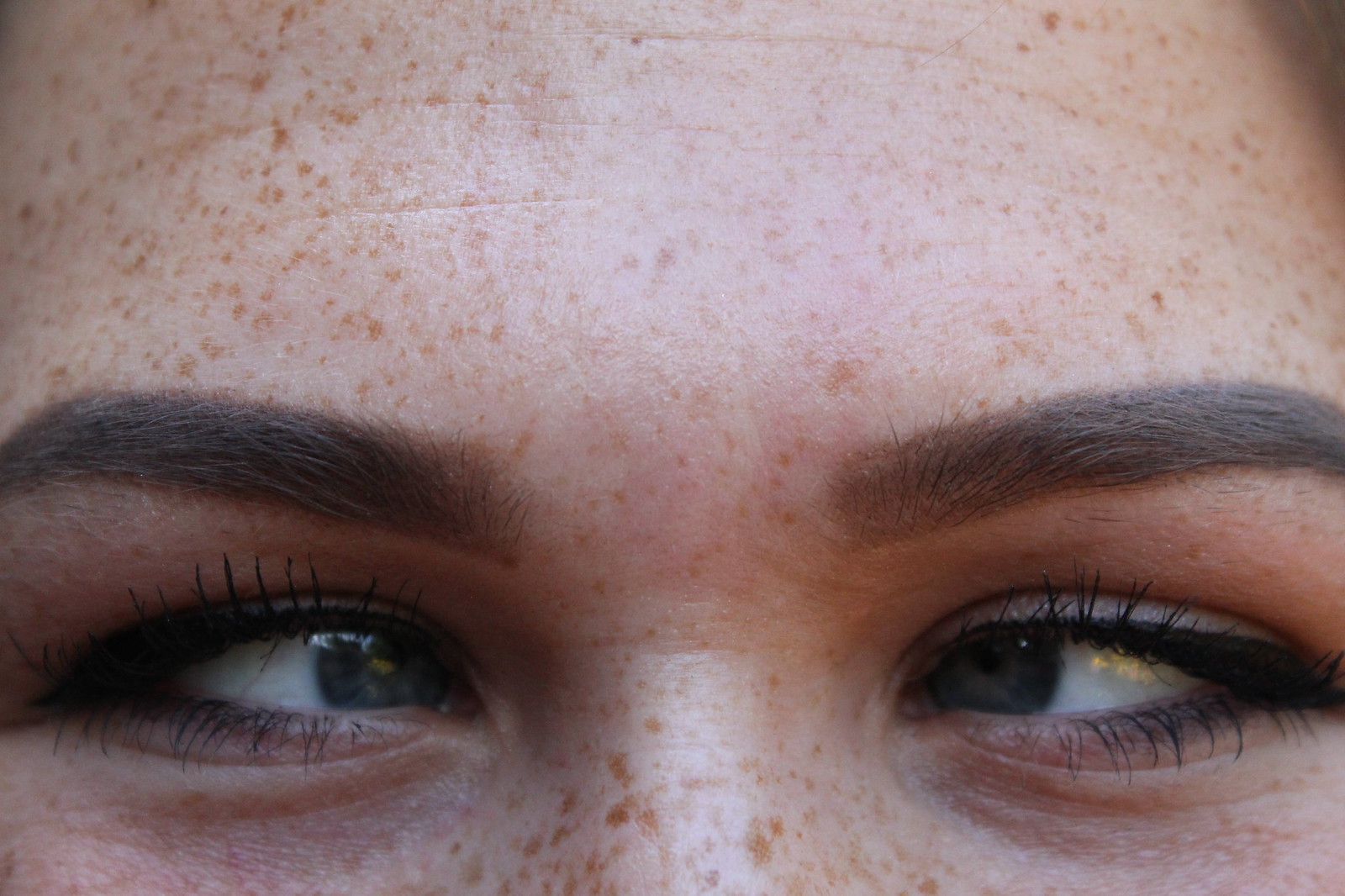This close-up image captures the face of a young Caucasian girl, focusing on her forehead, eyebrows, eyes, and the upper bridge of her nose. Her forehead is adorned with numerous tiny brown freckles, which continue across the visible portion of her nose. She has thick, dark brown eyebrows that frame her striking hazel eyes, accentuated by subtle black eyeliner and mascara on her lashes. Her eyes are pointed inward, creating a cross-eyed effect, and the whites of her eyes are clearly visible. Her forehead shows a few fine lines, and the photograph reflects natural daylight, suggesting she is outdoors.